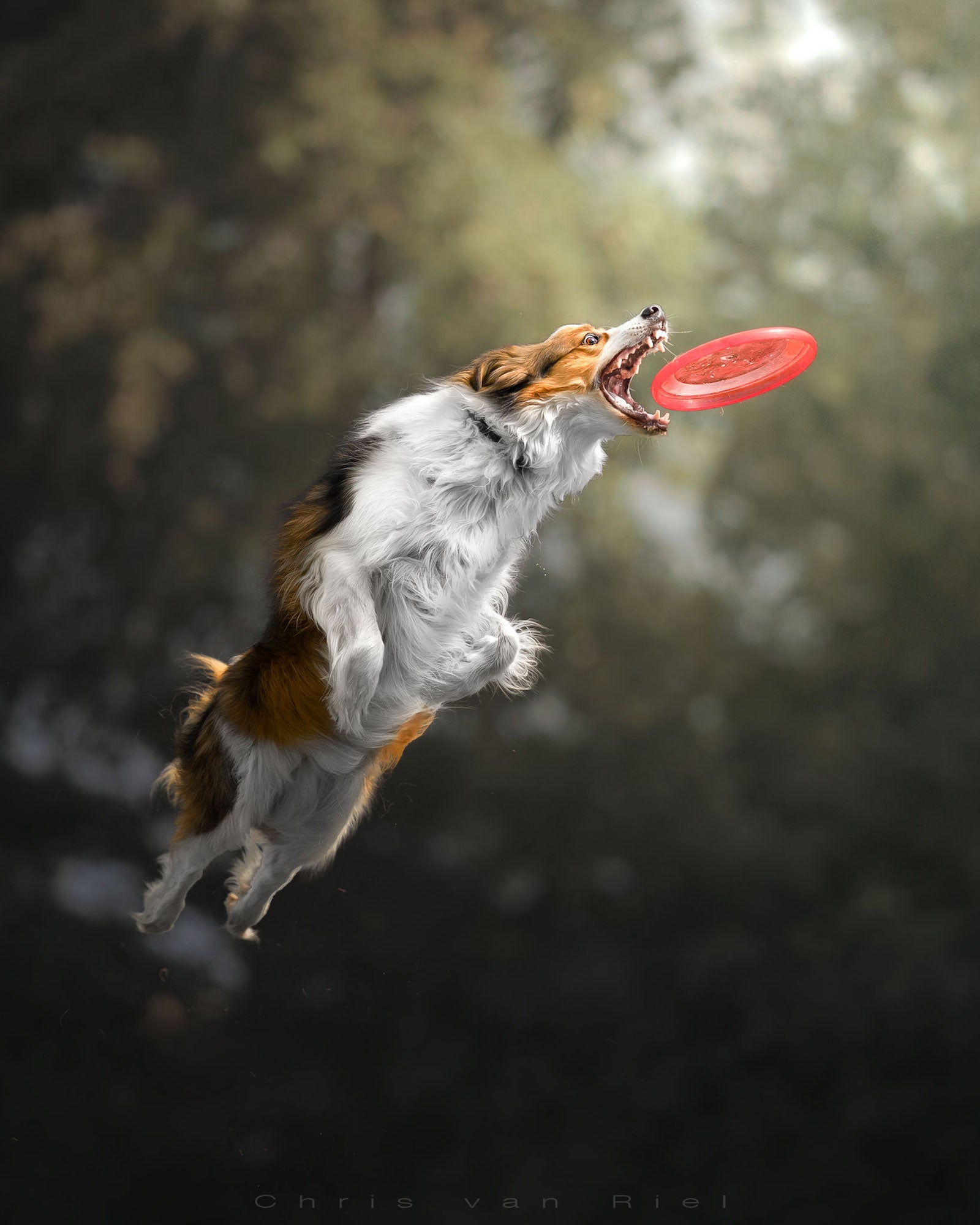In this dynamic outdoor action photograph, taken during the daytime with possible filter effects lending it a painting-like quality, we see a dog resembling a Shetland sheepdog or miniature collie, leaping midair with its mouth wide open, about to catch an orange-red frisbee. The dog, bathed in sharp focus against a blurred background of trees and bushes with light filtering through, showcases a distinctive coat: a white muzzle, chest, belly, and paws, coupled with light brown fur adorned with black spots. The dog's remarkably long neck appears almost stretched in the image. The artist, Chris Van Riel, has their name subtly inscribed in light grey at the darker bottom segment of the image, adding an elegant touch to this beautifully captured moment of canine agility.